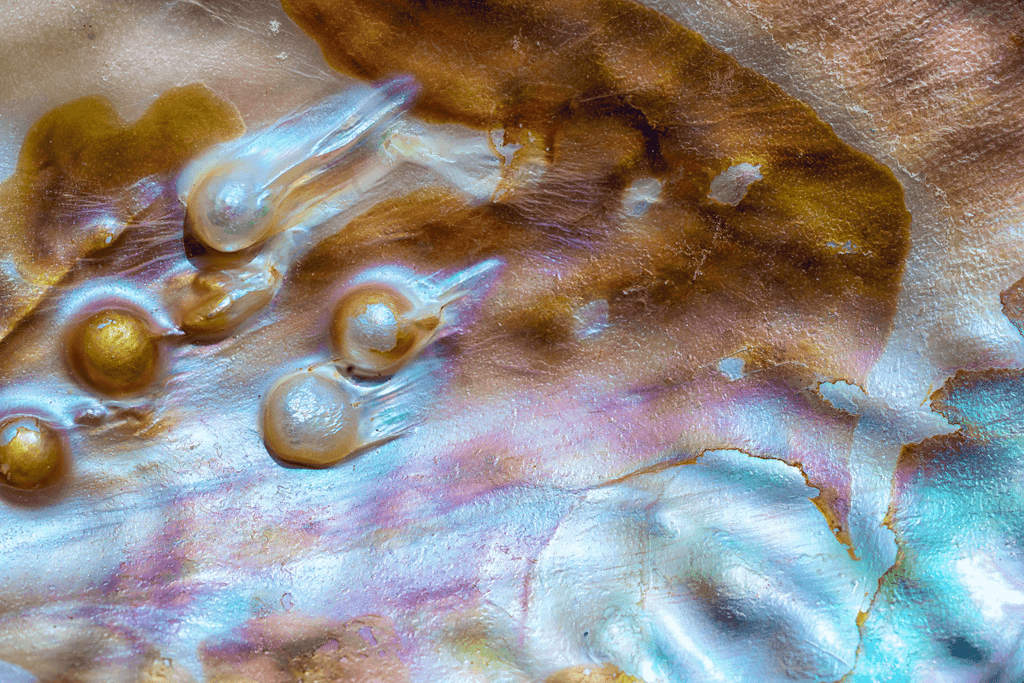The image showcases five pearls embedded within the iridescent, pastel-colored interior of a clam shell. The clam shell is rich in texture, adorned with a radiant blend of colors including natural gold, hazel brown, iridescent purple, and blue, further transitioning towards turquoise and baby blue on the right side. The overall surface appears smooth yet bumpy with irregular lines resembling brush strokes. The pearls are encapsulated in delicate gold shells, two of which are dark-colored gold and three are classic white. The setting evokes a tropical, island-like vibe, emanating a reflective, mother-of-pearl glow and creating a visually captivating scene that blends art with nature’s craftiness.